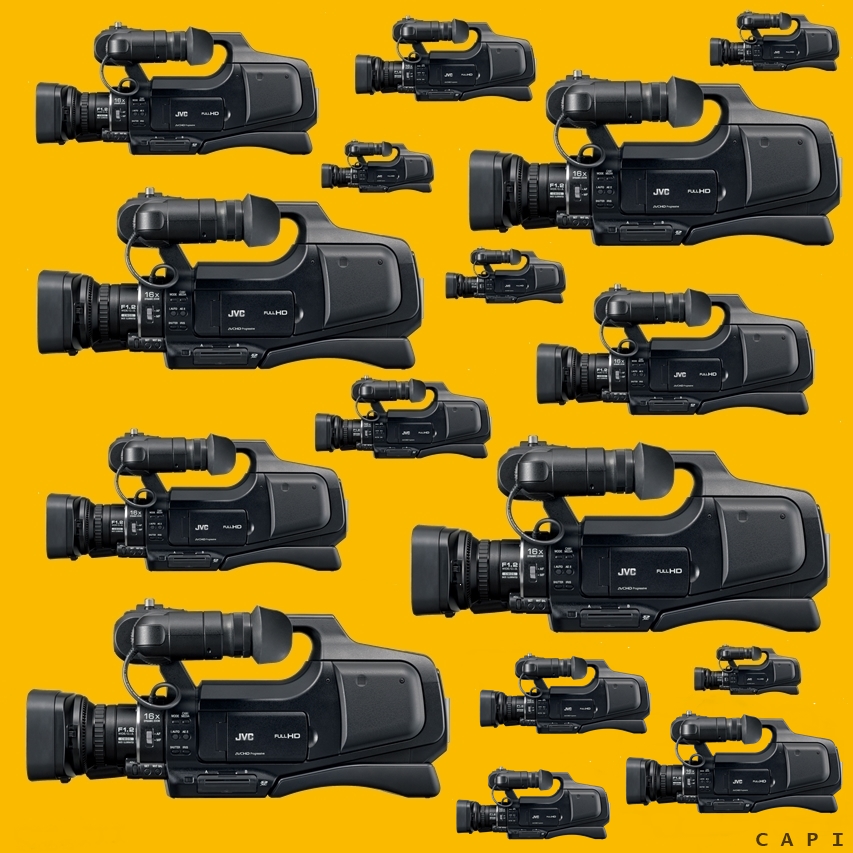The image is a vibrant, digitized composition featuring approximately 16 JVC video cameras of varying sizes, all with the lens facing left against a striking yellowish-orange background. The cameras are scattered across the entire image surface, with some being large, others medium, and a few small and extra small. Each camera displays the logo "JVC" and the text "Full HD," with lenses marked "16X." Visible cords curl from the tops of the cameras onto their lenses, and a light source shines on them, adding depth and dimension. In the lower right corner of the image, the initials "CAPI" are prominently displayed, possibly indicating the creator of the artwork.